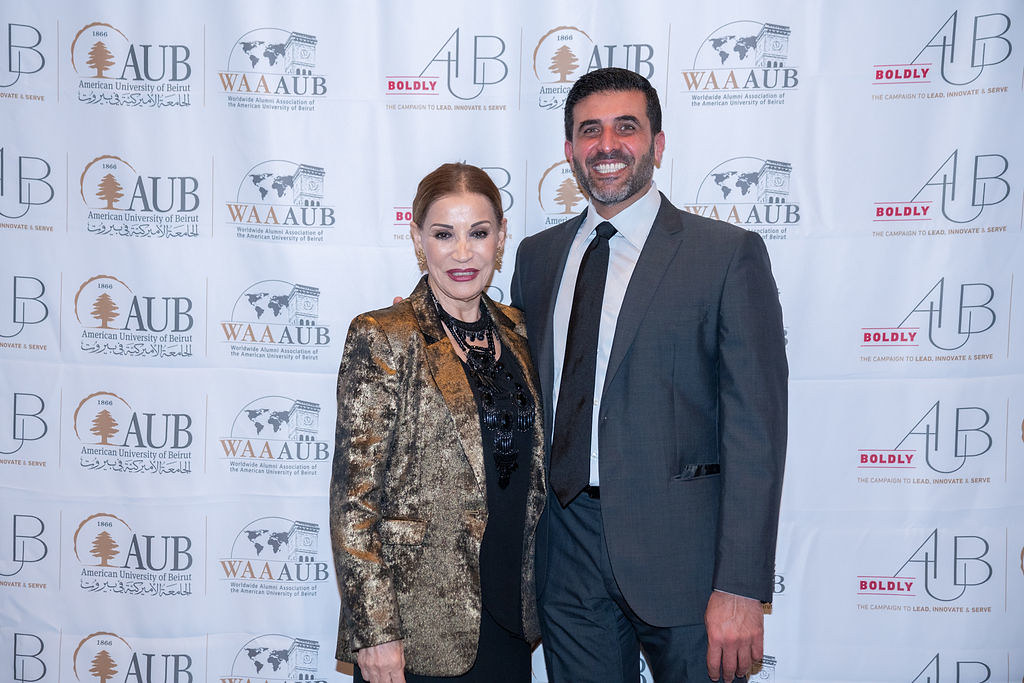The photograph captures a well-dressed couple standing arm-in-arm at an event, posing in front of a backdrop filled with repeating logos. The backdrop is predominantly white and features several logos including "AUB" in silver letters, "American University of Beirut," "WAAAUB," and the word "Boldly" in a bold, stylized font, along with some Arabic text and illustrations, such as a tree and a tower with a clock set against a world map.

On the left, there's an older woman with light brown hair styled back in a bun. She is elegantly dressed in a gold velvet blazer over a black shirt or dress, accessorized with a prominent black necklace and matching gold earrings. She is wearing well-applied makeup, including red lipstick and drawn-on eyebrows, and smiles at the camera. Beside her, on the right, stands a middle-aged man with short black hair and a beard. He is dressed in a gray suit jacket, paired with a white shirt and a gray tie. The two have their arms around each other's shoulders or lower back, highlighting their close relationship.